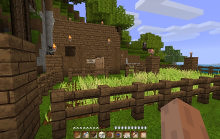A small screenshot from the game Minecraft, likely featuring some modifications as indicated by the altered heads-up display (HUD). The image showcases elements distinct to the popular sandbox game, reflecting the player's personalized or modded experience.